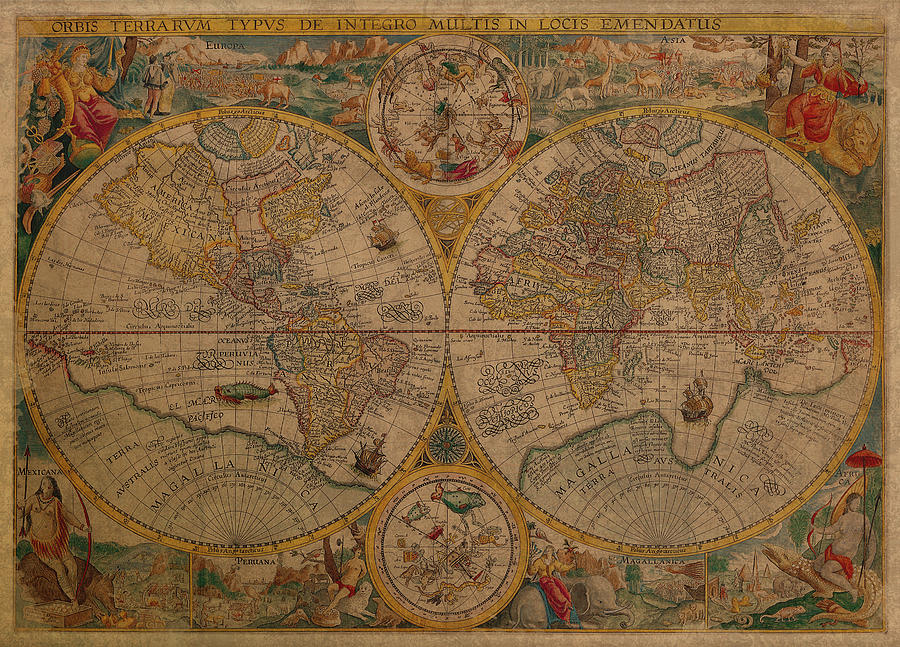The image is a highly detailed, vintage map from 1599, featuring two large, circular representations of the world in dark and light brown tones. The left circle appears to depict North and South America, while the right circle showcases Europe, Asia, and Africa. The continents are not perfectly shaped as we envision them today, suggesting it's a historical or artistic interpretation of the world. A yellow banner at the top contains dark writing in a language that resembles Latin, stating, "Orbis Terra Vroom T Y P V s de integro Multi in locus."

Surrounding the circles are smaller circles, possibly compass roses, and intricate illustrations, including biblical-like goddesses similar to the art in the Sistine Chapel. The map is adorned with various drawings of people, animals—like elephants and rhinoceroses—and ships, adding to its ornate and decorative appearance. One striking image shows a man sitting on a reptile, blending reality and mythology. Additional text labels regions such as "Mexicana," "Peru Vanna," and "Magellanica," further enhancing its historical richness.

This map is not only a cartographic representation but also a piece of ancient art, filled with symbolic and decorative elements, showcasing the cultural and artistic sensibilities of its era.